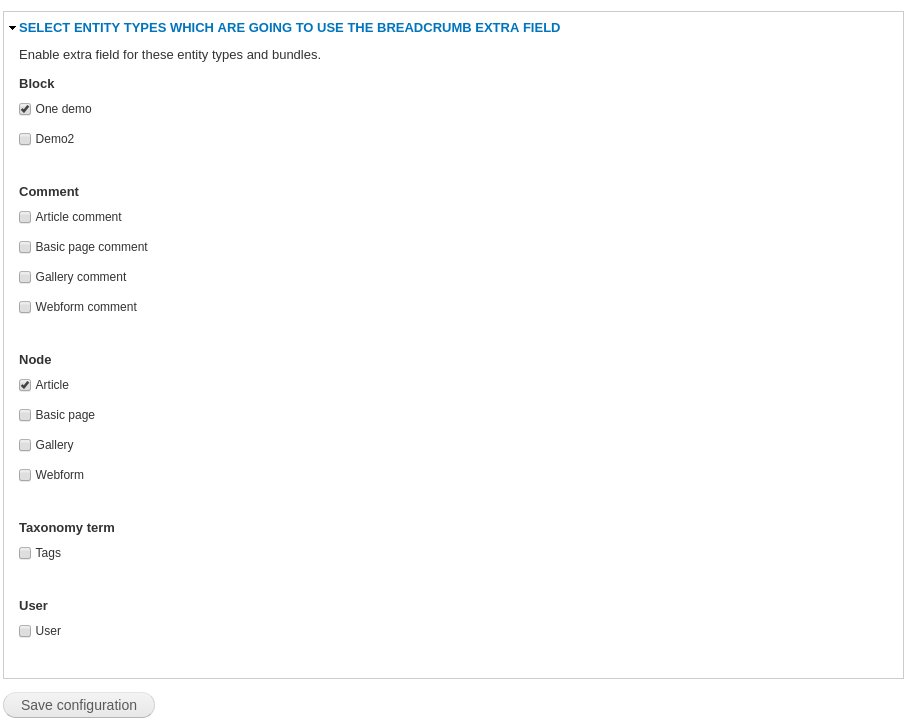The image depicted is a configuration screen for selecting entity types that will utilize an extra breadcrumb field. The page contains a well-structured list composed of several sections with corresponding subcategories. Here's a detailed breakdown:

At the top of the page, there is a blue header that reads: "Select entity types which are going to use the breadcrumb extra field."

Below this header, the content is displayed in black text on a white background. It begins with the section title: "Enable extra field for these entity types and bundles."

The main content is categorized into five segments, each section featuring checkboxes aligned to the left, with explanations and choices on their right. The details are as follows:

1. **Block**:
    - Two choices available, with one selected:
        - Demo 1 (Chosen)
        - Demo 2

2. **Comment**:
    - Multiple choices available, none selected:
        - Article Comment
        - Basic Page Comment
        - Gallery Comment
        - Web Form Comment

3. **Node**:
    - Four choices available, with one selected:
        - Article (Chosen)
        - Basic Page
        - Gallery
        - Web Form

4. **Taxonomy Term**:
    - One choice available, none selected:
        - Tags

5. **User**:
    - One choice available, none selected:
        - User

At the bottom left of the page, there is a button labeled: "Save Configuration," indicating that no changes have been saved yet.

This screen appears to be part of a user interface, where users configure which entity types will utilize additional breadcrumb fields, making it a feature-rich, yet currently unsaved, configuration process.